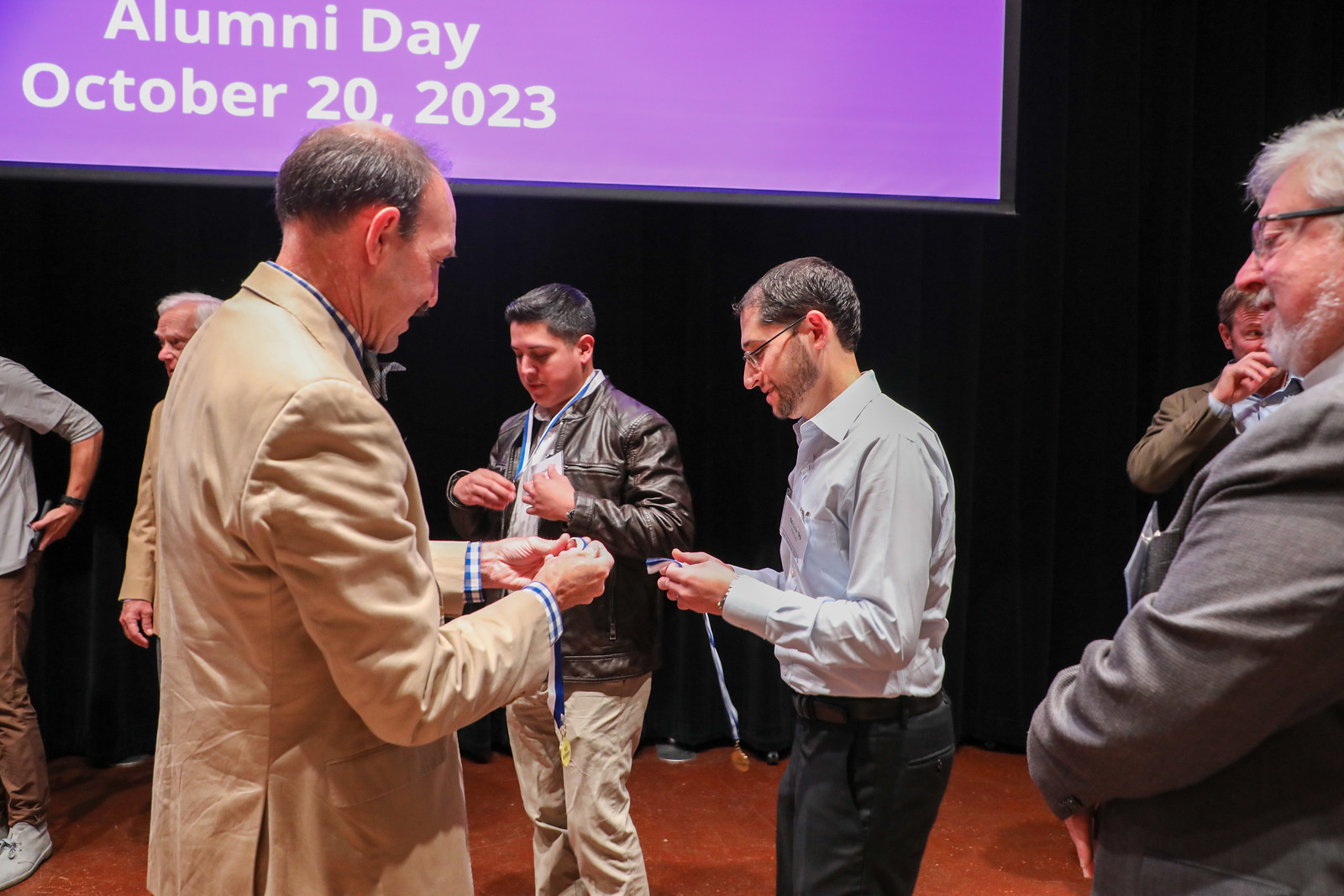The photograph captures several men dressed in business casual attire, standing on a brown-floored stage with a black curtain backdrop. They are actively putting on lanyards or necklaces. The men are not facing the camera but are instead looking in various directions at each other. In the upper left-hand corner of the image, there is a projector screen with a purple or red background displaying the text "Alumni Day, October 20th, 2023" in white. The entire image is horizontally oriented, with the group of men centered towards the bottom half, suggesting an indoor event setting, possibly a school reunion. The color palette includes tones of purple, black, gray, beige, blue, tan, and brown.